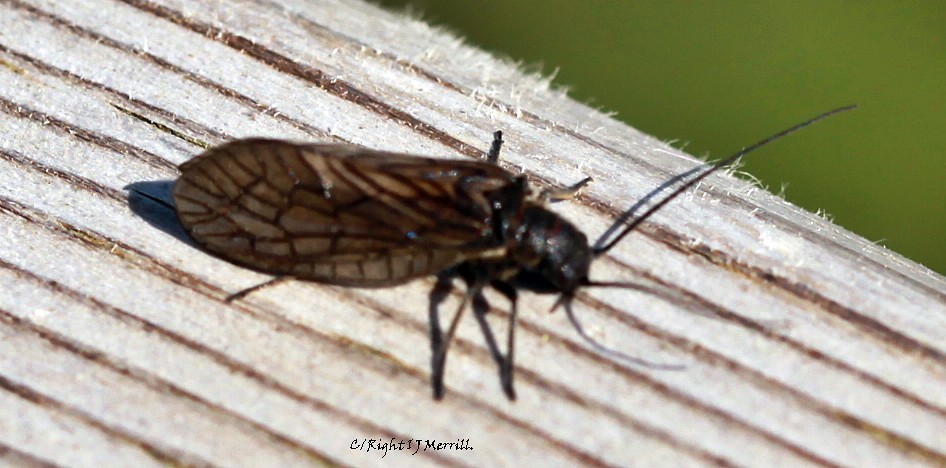The image depicts a black winged insect, possibly a cicada, resting on a light brown wooden surface that has diagonal grain patterns running from the left-hand corner to the right-hand corner. The wood's texture is clear, with rough, fuzzy patches that accentuate its natural look. The insect has two large, translucent wings with dark veins that give them a stained glass appearance. It's positioned near the top center of the picture where the wooden background transitions into a dark olive green area, possibly indicating an outdoor setting with grass or foliage. The cicada casts distinct shadows from its body, legs, and long antennae, which spread outwards. Below the insect, there is a partial, unclear text reading "C / writes IJ Merrill." Six legs are visible, and the overall color of the insect and wooden surface appears enhanced by sunlight, highlighting the scene’s natural details.